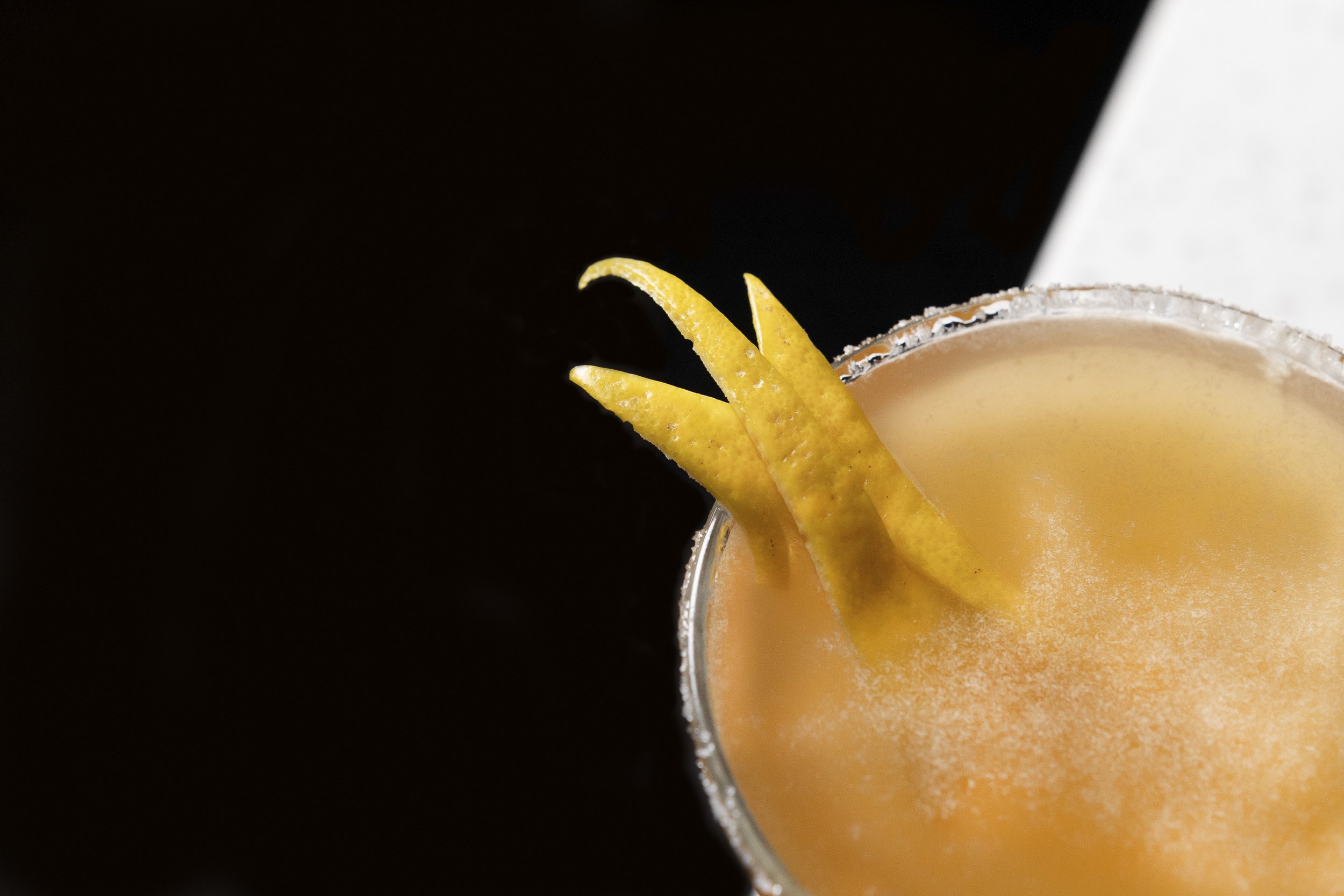This photograph features a close-up of a round, clear glass cup positioned towards the bottom right side of the image. The cup contains an orange-colored liquid, likely an icy blended drink, with a texture resembling mesh ice. The rim of the cup is garnished with white sugar. Emanating from the liquid are three yellow, arm-like extensions that resemble octopus arms, likely lemon peels. Scattered at the surface of the drink are white sprinkles. The background of the photograph consists of a stark contrast between a majorly black area covering the left side extending up to the right of the cup, and a white area occupying the top right corner, framing the intriguing focal point of the cup and its contents.